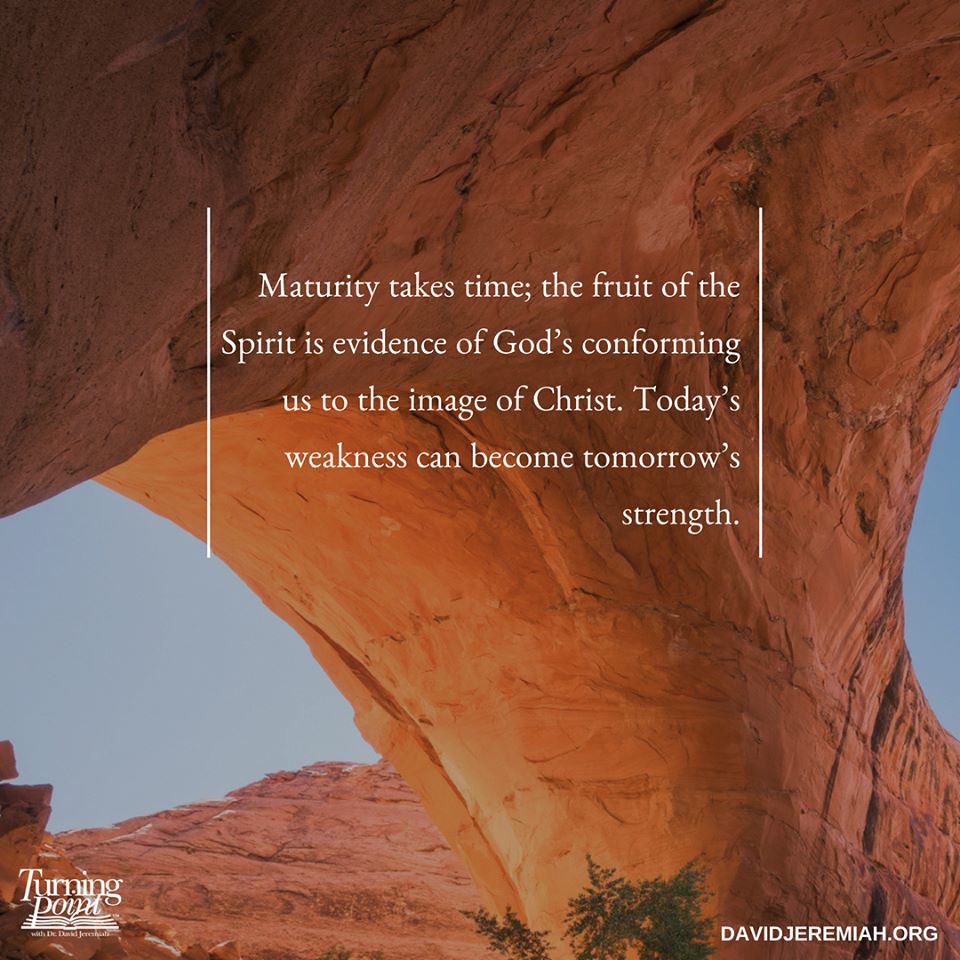This outdoor image depicts a massive, textured, pink-orange rock archway, likely found in a desert landscape reminiscent of Arizona or the Grand Canyon. The rock formation includes areas lit by sunlight and shaded pockets, enhancing its rugged beauty. Through the archway, the clear blue sky and additional red-orange rock formations can be seen in the distance. Sparse vegetation is visible at the bottom of the scene. Overlaid on this stunning natural backdrop is an inspirational quote in white text, centered within vertical white lines. It reads, "Maturity takes time. The fruit of the Spirit is evidence of God's conforming us to the image of Christ. Today's weakness can become tomorrow's strength." In the bottom left corner, the caption "Turning Point" appears alongside an open book icon, while the bottom right corner bears the website "DavidJeremiah.org."